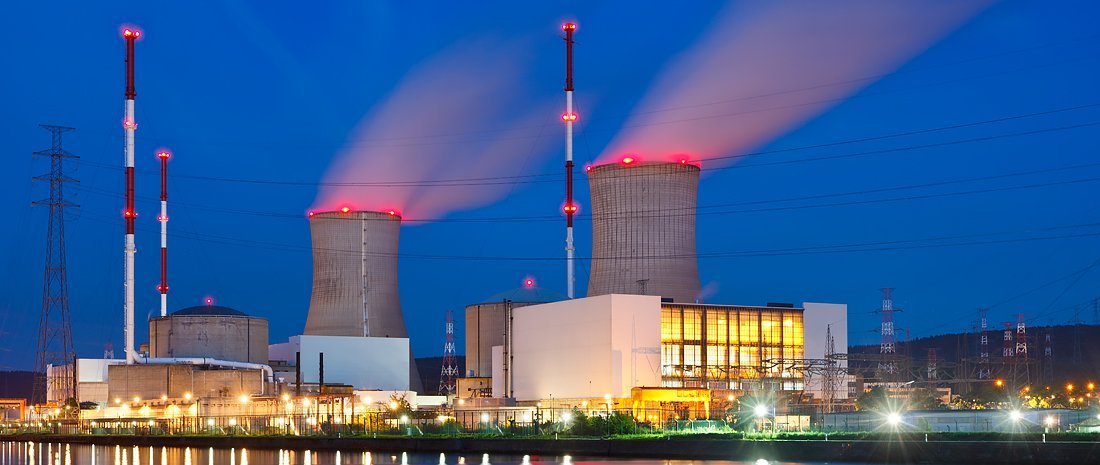This professionally taken, horizontal color photograph captures a modern nuclear power site at twilight. Dominating the scene are two monumental nuclear cooling towers, their upper rims adorned with red lights and emitting plumes of steam. In front of the nearest tower stands a brightly illuminated, multi-windowed building. To the left of this, there is a smaller cement tower and another smaller cement building. The photograph's background is dotted with numerous towering structures, including electrical towers strung with power lines spanning the width of the image. The far left of the frame features a particularly tall electric tower. The thin strip of water at the bottom left reflects the ambient lights, adding to the vibrant blue hues of the dimming sky. The site is well lit with numerous lights lining pathways around the facility, ensuring visibility and safety for nighttime operations.